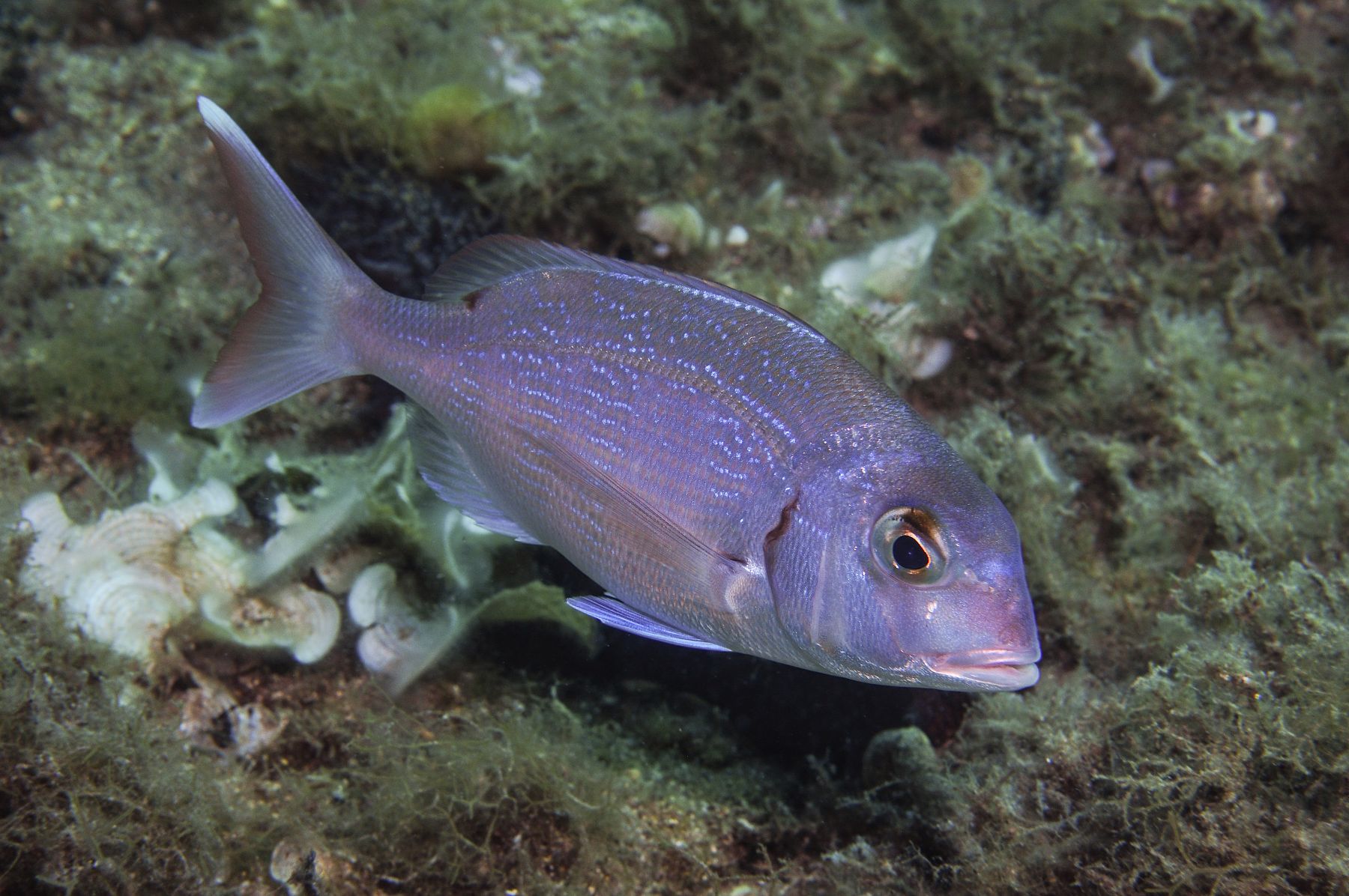This color photograph, taken in landscape orientation, depicts a purplish-blue snapper swimming near the bottom of an ocean or lake. The fish, which features light blue speckles along its elongated body, occupies more than half the width of the image. Its position, with its tail facing the top left and its head facing the bottom right, reveals a short dorsal fin and a slightly open pink mouth. The snapper’s large golden eye with a black center is looking up at the viewer. Below the fish, the seafloor is scattered with green seaweed or algae and a few white shells concentrated on the left side. The underwater scene includes ferns and coral formations, with more green algae visible in the upper left and right corners. The style is realistic underwater photography, capturing the solitary fish in its serene, natural habitat.